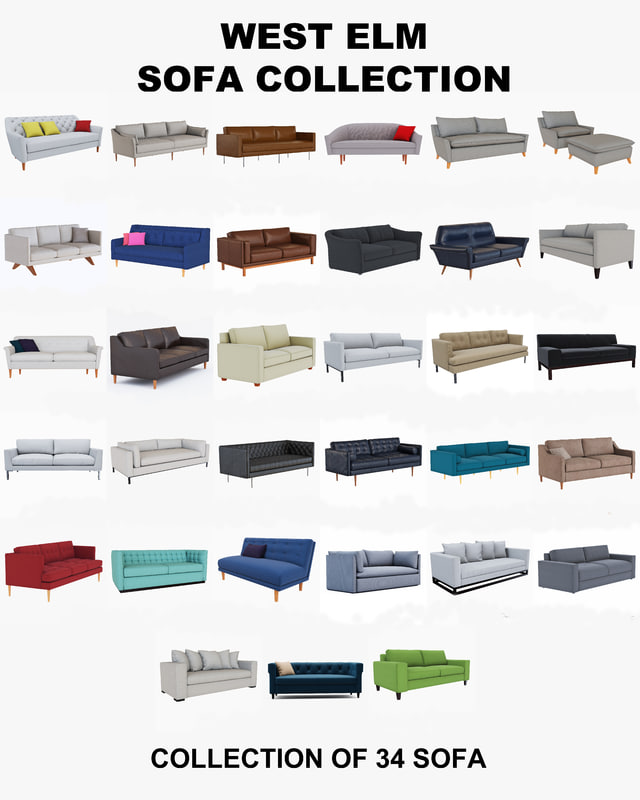This is an advertisement for the West Elm Sofa Collection, prominently displayed against a very light lime background. The top of the image features the text "West Elm Sofa Collection" in bold black letters. The bottom of the page reads "Collection of 34 Sofa" in black text, although there are actually 33 sofas depicted. The sofas are arranged in a neat collage, with six sofas per row for the first five rows and three sofas in the last row. Each sofa varies in color and style; notable colors include whitish, brown, black, blue, red, and green. Most sofas are two or three-seaters, many featuring little legs while a few sit flat on the ground. Some sofas face left, others right, adding visual diversity. The last row consists of a gray, a brilliant blue, and a green sofa. Additionally, some sofas are accessorized with throw pillows in colors like yellow, red, and pink, adding to the overall vibrant display.